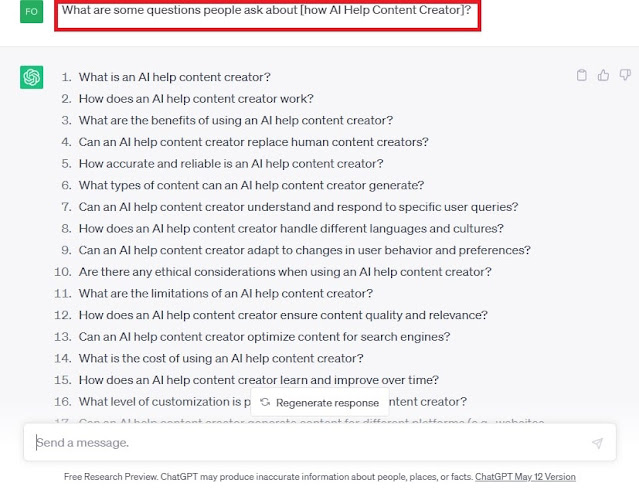The image is a screenshot of an AI chatbot interface, specifically Chatbot GPT. At the top of the image, a search bar is highlighted with a red rectangle, and within this bar, the phrase "What are some questions people ask about (how AI help content creator)?" is prominently displayed. Adjacent to the search bar on the right side is a green box labeled "FO."

Below the search bar, a list of 16 questions is shown, though the list appears to be cut off at the bottom. The first four questions in the list are visible and include:
1. What is an AI help content creator?
2. How does an AI help content creator work?
3. What are the benefits of using an AI help content creator?
4. Can an AI help content creator replace human content creators?

The image effectively illustrates common inquiries related to AI's role in aiding content creators, providing a snapshot of typical user interests and concerns in this domain.